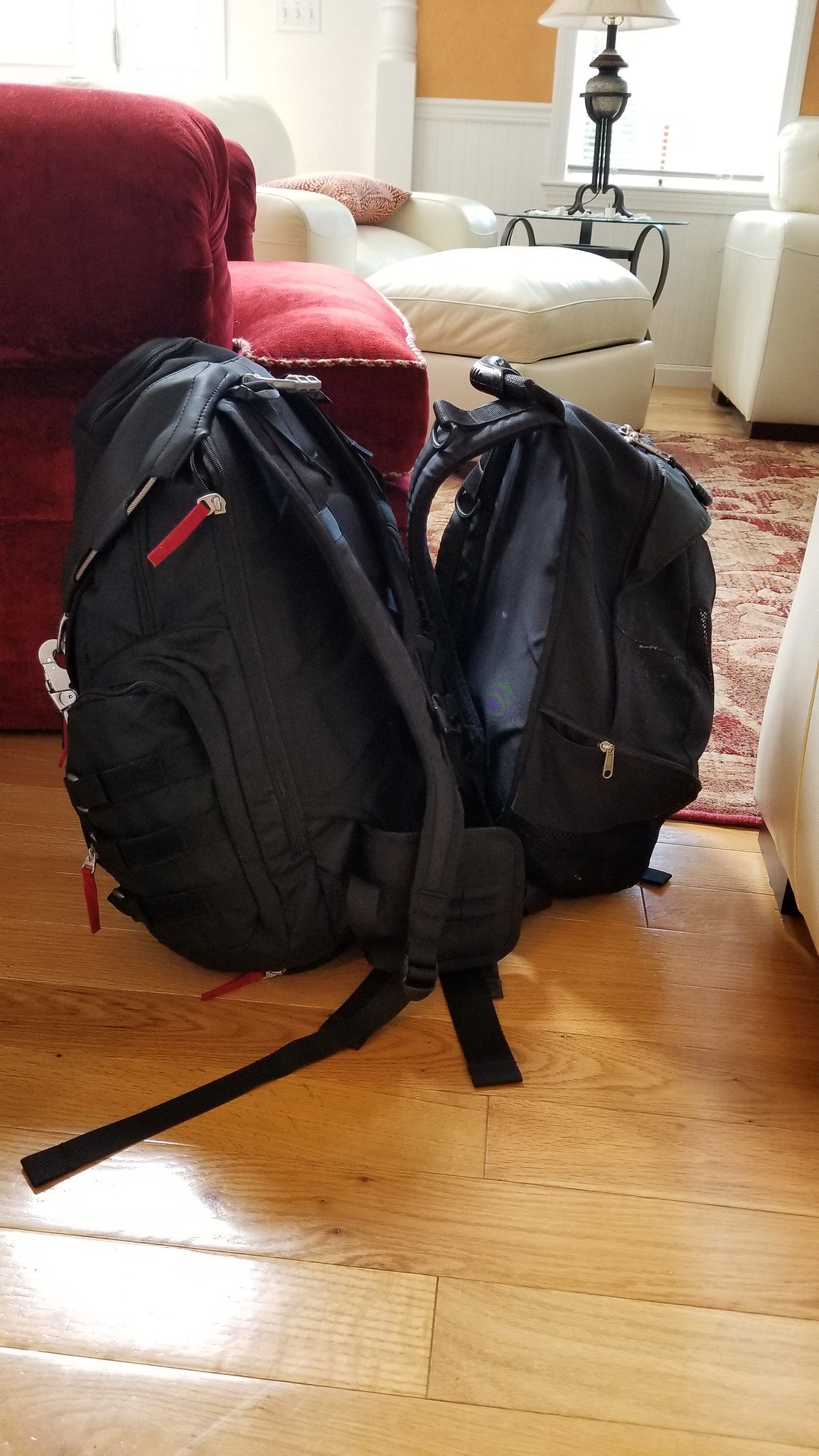The image depicts two backpacks, one black and one blue, standing upright and tied together by a red intricate V-designed rope strung through their top handles, creating tension that keeps them balanced. They rest on a light brown wooden floor in a well-lit living room. In the foreground, there's a vibrant red couch directly behind the backpacks, while further back, a white couch and a white ottoman subtly frame the scene. The left backpack is predominantly black with red tassels on its zippers, larger than its blue-accented counterpart. The natural light streaming in from two windows illuminates a side table and mirror in the distance. The room exudes a cozy, lived-in charm, punctuated by the detailed textures and colors of the furniture and the unique arrangement of the backpacks.